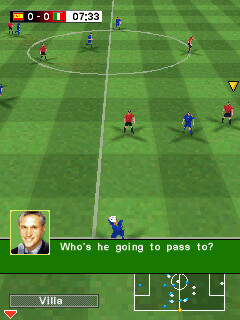This image is a screenshot from a soccer video game, capturing an intense moment on the field. The field is designed with large squares alternating in shades of light green, dark green, and medium green. The score, located in the upper left corner, is tied at 0-0, accompanied by two flags representing the competing teams and a game time display reading 07:33. 

The players are divided into two teams, one wearing red shirts and the other wearing blue shirts. At the bottom of the screen, towards the left-hand side, there's an image of a man with the caption, "Who's he going to pass to?" This suggests a decision-making moment in the game. A player in a blue shirt is positioned at the bottom of the screen, poised to throw the ball.

In the bottom left corner, the name "Villa" appears with a red triangle pointing down beneath it. To the right, there is an overhead view of the field showing the current positions of the players, who are represented as colored dots. A yellow arrow highlights one of the players in a red shirt, located towards the center of the field, indicating a potential pivotal play.